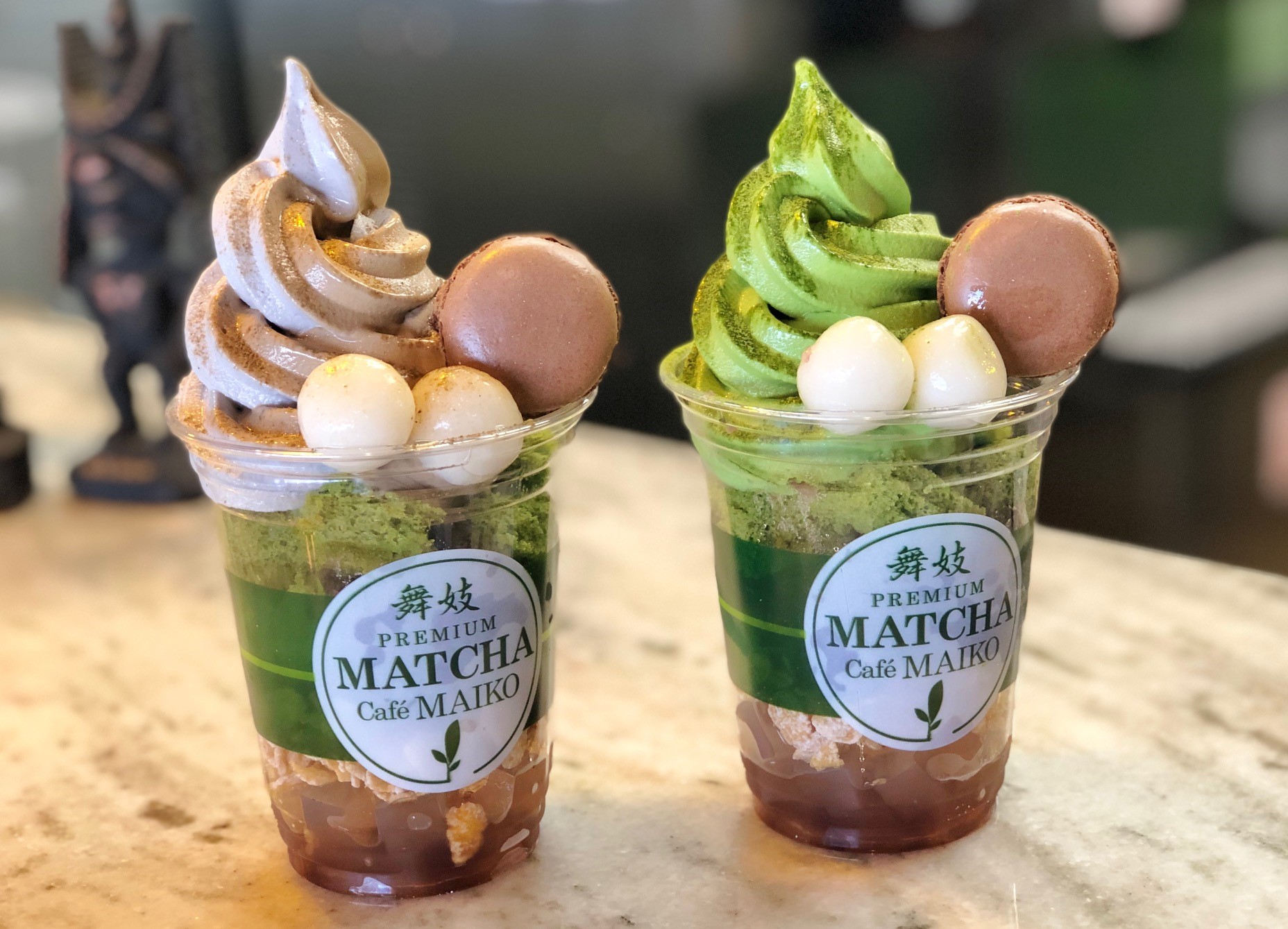The image shows two transparent plastic cups, placed on a light brown wooden surface, and each cup is labeled with the text "Premium Matcha Cafe Maiko." The labels feature green bands with white circles that encase green leaves and the cafe's name. Both cups appear to contain layered desserts with a variety of colors and ingredients. Near the bottom, the content in each cup is brown, possibly indicating a coffee-based substance or a different type of dessert. 

As you move upwards, green and white elements become more apparent. One cup contains a swirl of green ice cream, likely matcha-flavored, while the other cup features a swirl of brown ice cream. Complementing these ice creams are white balls that resemble tapioca pearls or similar dessert components, as well as brown, cookie-like items. Additionally, both cups have some small round elements which could be ice cream balls or other sweet treats, making the overall appearance intricate and visually appealing, possibly suggesting a rich, multi-layered dessert.